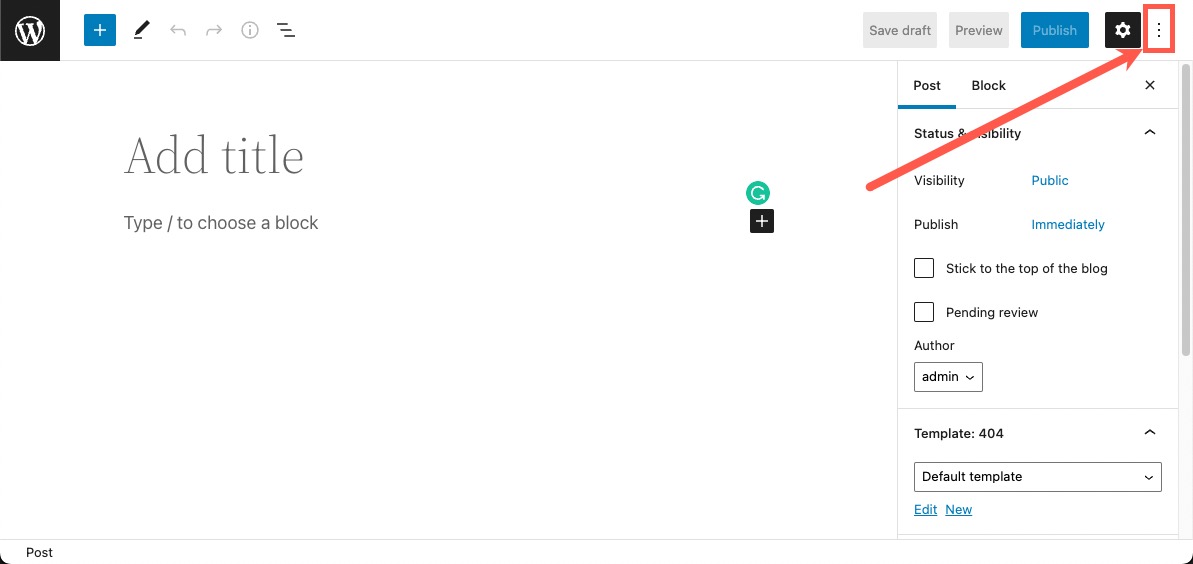The image showcases a well-designed website interface, predominantly featuring a sleek black header. Centered within the header is a black logo encircled by a thin white ring, housing a white "W" at its center. Adjacent to the logo is a plus button, and icons allowing for various actions such as writing, navigating backward and forward, and accessing the internet. Notably, a customized hamburger menu icon resembles a backslash.

On the right side of the header, options like "Save Draft," "Preview," and "Publish" are available, with "Publish" prominently displayed against a blue background, unlike the others which have grey backgrounds. Additionally, a settings button and a three-dot menu are present.

The main body of the interface prompts the user to add a title and to type or choose a block for their content. A sidebar on the right offers further functionalities including toggling between "Post" and "Block" modes. Currently, it is in "Post" mode, displaying detailed options under "Status and Availability." These settings show that the post's visibility is set to public, it can be published immediately, stuck to the top of the blog, or marked as pending review. The author dropdown menu is set to "admin," and the template dropdown, currently showing "Template 104," has a default template selected.

At the bottom of the sidebar, users have the option to post their content once they are ready. This detailed, user-friendly interface is designed to streamline the content creation and publishing process.